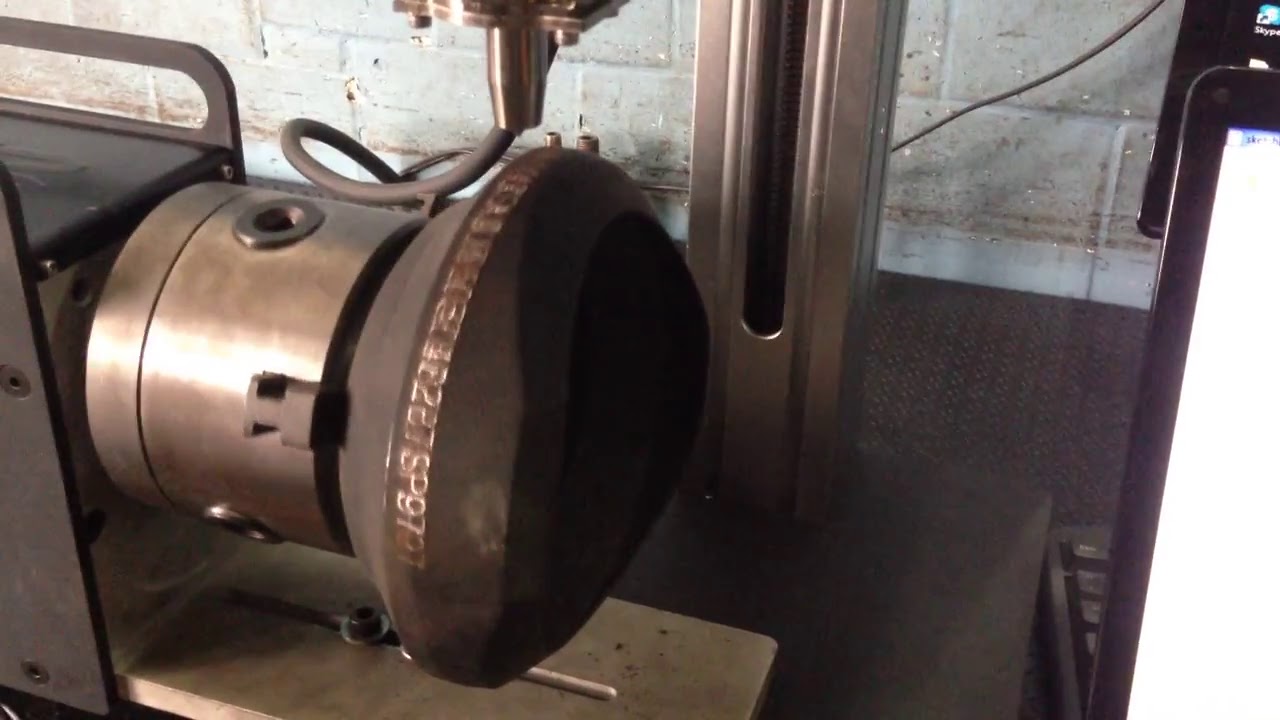The photograph depicts a metallic machine, predominantly grey or silver, featuring a motor and a rotating component. Attached to this machine is a cylinder with a mushroom-like cap, which has a black knob jutting out. Around the edge of this knob, there are series of stamped letters and numbers, including "227SP97" in a gold font. The cylinder is connected to a larger frame by a pipe or hose, suggesting it is part of a more complex setup. The machine is mounted on a dark grey metallic surface, and the setting includes a background wall, which appears somewhat dirty. There is a slight inconsistency in the wall's description, ranging from light blue to cream to rustic grey, indicating possible variations in lighting or wall condition interpretation. The ground is dark grey, and numerous nuts and bolts can be seen at various points on the machine, adding to its intricate, industrial appearance.